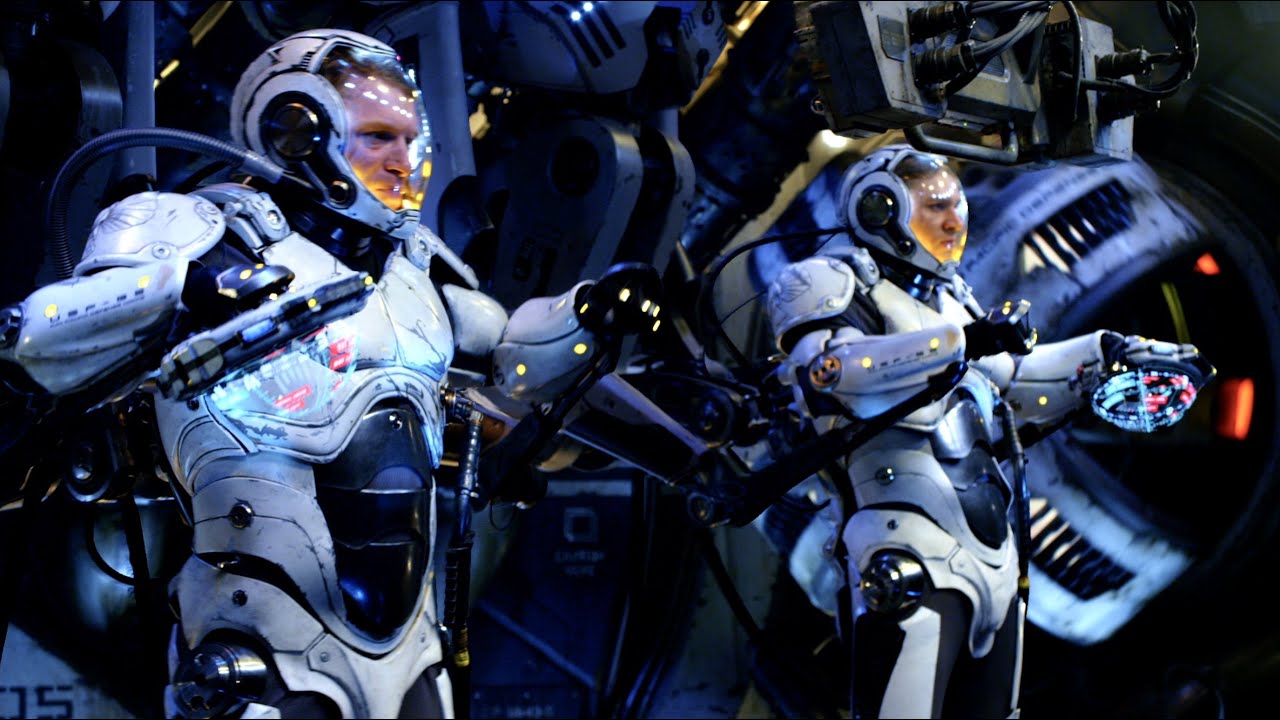The photograph depicts a scene likely derived from a futuristic sci-fi movie, showcasing two astronauts outfitted in advanced, form-fitting exoskeleton suits reminiscent of Iron Man or Pacific Rim mecha pilots. The suits are primarily white with black detailing and feature clear visored helmets, allowing the faces of the male astronaut on the left and the female astronaut on the right to be visible. The astronauts appear to be in their thirties, each extending their arms slightly to manipulate controls. Behind them, metallic structures and coils provide support, mimicking an Android exoskeleton. Both are intently focused on a holographic screen in front of them, which may provide essential information or controls for their environment. The background is shrouded in darkness, adding to the intense and futuristic ambiance of the scene. The astronauts' helmets are equipped with tubes, likely supplying oxygen, and they exhibit blank, concentrated expressions as they engage with the machinery.